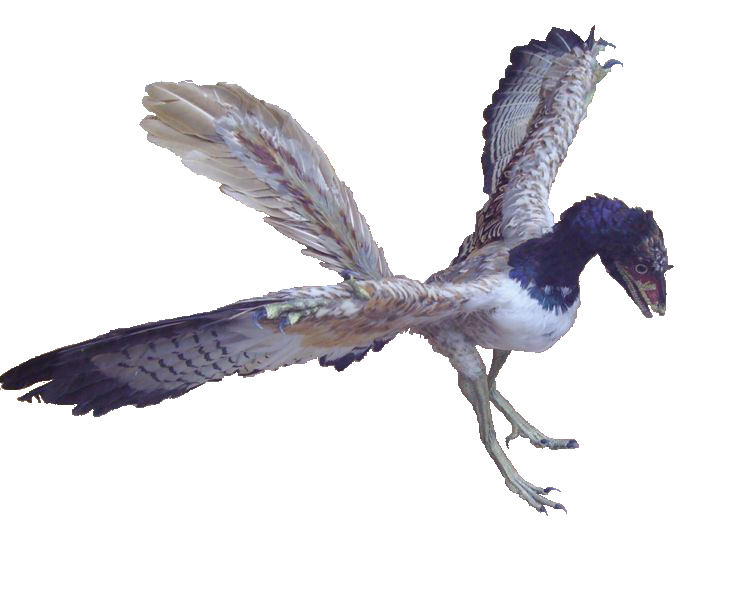This image features a striking bird with its wings outstretched against a stark white background, showcasing its intricate plumage. Its head is predominantly black, accented with vibrant red around the facial area, giving it a distinctive appearance. The bird's eyes are a captivating white set against black pupils. Its breast is white, contrasting with the variegated brown and white feathers that adorn its wings. The tail feathers exhibit a combination of brown and white, with a prominent black strip running through. The bird's sharp talons are notably black, and its legs white, adding to the overall striking color palette that includes hints of blue and beige around the wing and tail edges. The creature's head and neck transition into a subtle blue near the beak area, creating a fascinating blend that hints at its prehistoric, dinosaur-like heritage. This bird’s intricate coloring and fierce talons give it a unique, almost mythical appearance.